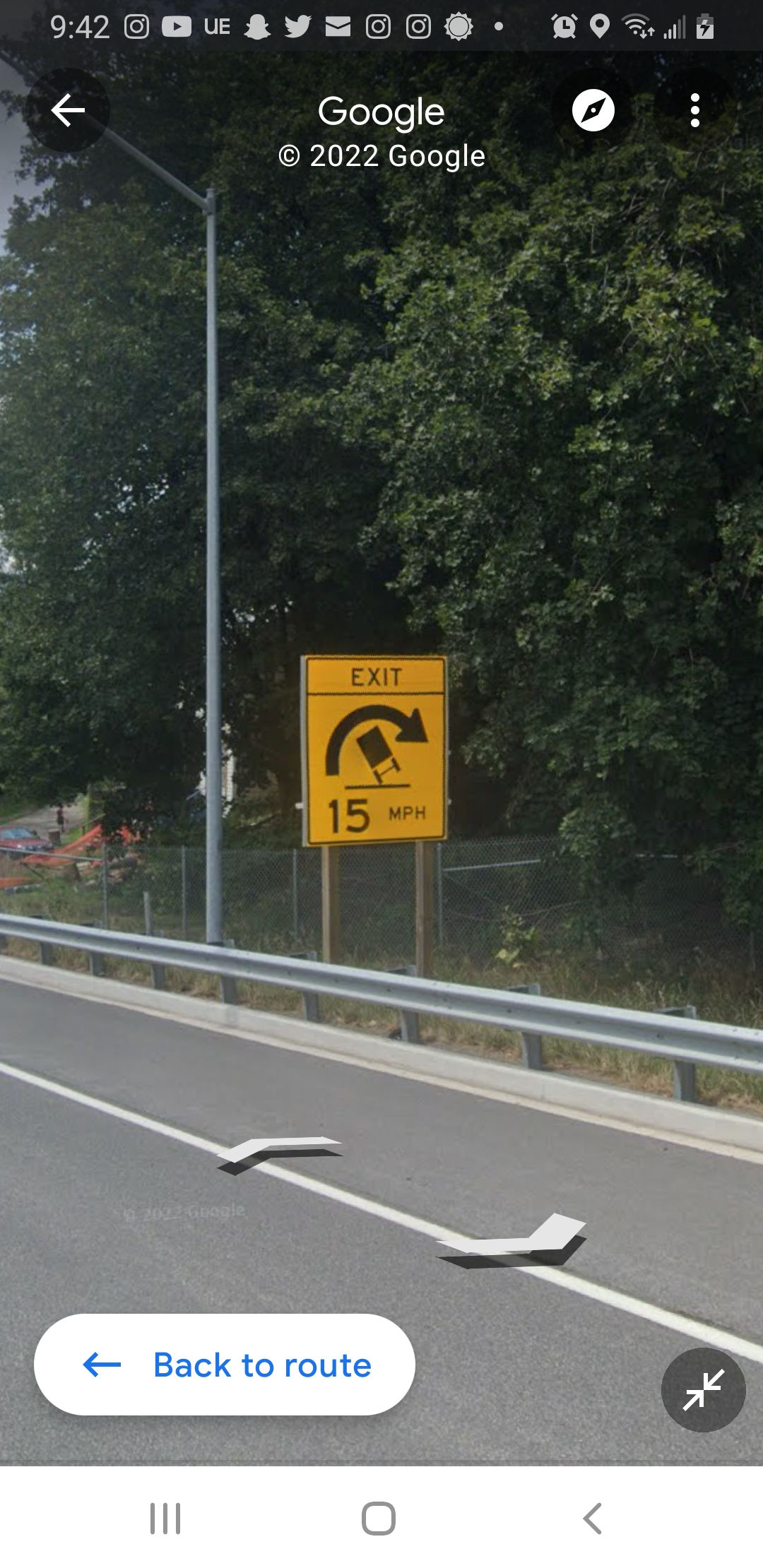This is a detailed screenshot taken on a phone of a Google Maps street view image. The image is vertical and at the very top, a black bar displays various app icons like Instagram and YouTube, the current time on the top left, and signal information on the top right. Just below this bar, it says "Google, copyright 2022 Google." To the left of this text, there is a back arrow inside a circle, and to the right, a directional icon and three vertical dots for more features.

The main Google Maps image shows a roadway with two large directional arrows: one pointing north and the other south, indicating possible movement directions. On the road's shoulder, there is a white line and a silver guardrail partially visible in the bottom left corner. Prominently in the center of the image, a yellow caution sign warns drivers about a sharp corner that must be taken at 15 miles per hour; it also features an image of a truck tipping over.

At the bottom left of the image, a white button with the text "Back to Route" and an arrow icon provides a navigational option. In the lower right corner, there are two arrows facing each other for minimizing or maximizing the image. The bottom of the screenshot also shows typical phone navigation buttons - three horizontal lines on the left, a circle in the middle, and a left-facing arrow on the right. The overall screenshot illustrates a side road view with clear navigational instructions and warnings.